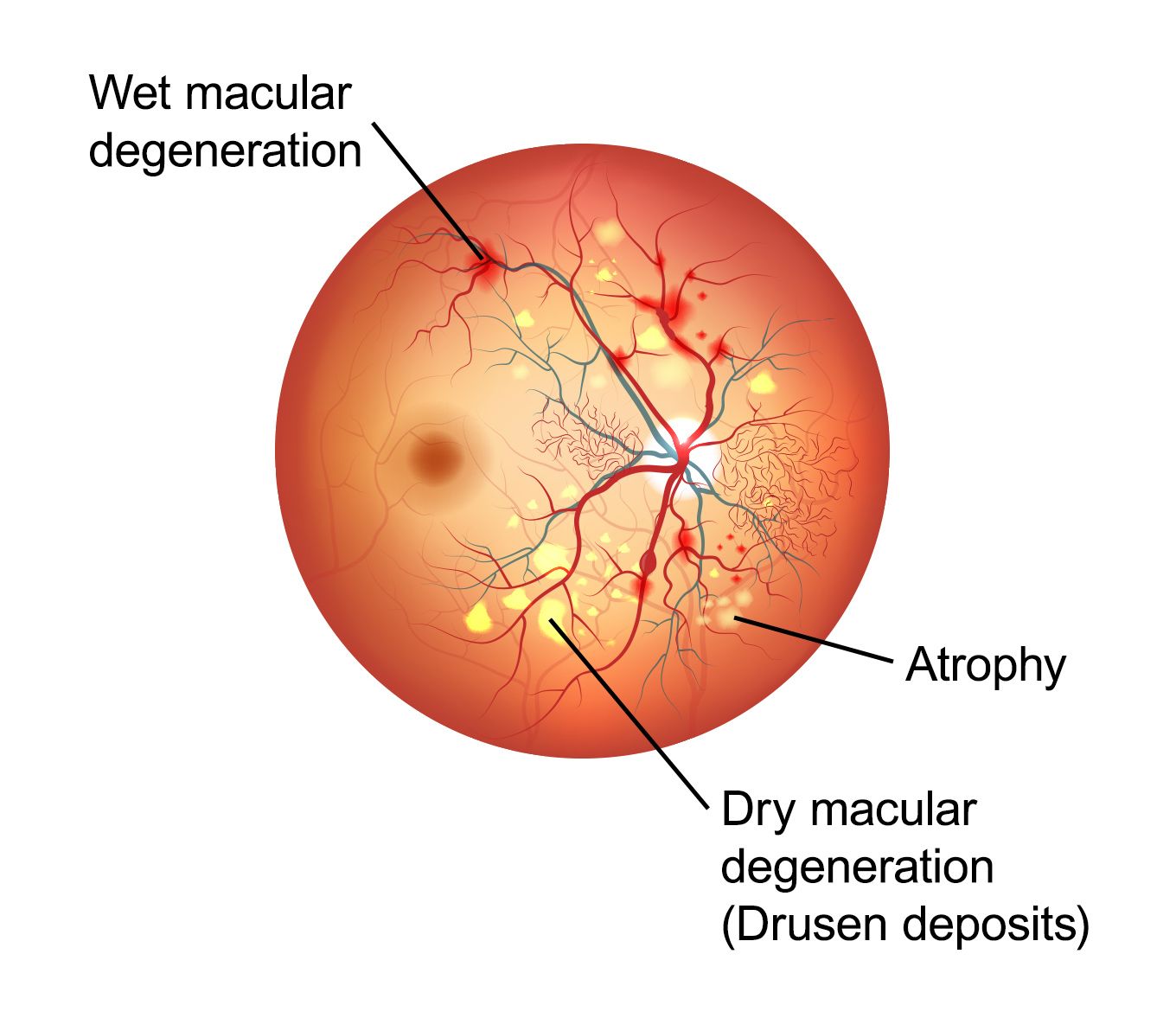This square, color illustration presents a detailed, computer-enhanced diagram of an eyeball, depicted from the back side, with the pupil not visible. Set against a plain white background, the central spherical object is shown in a vivid red and orange palette, highlighting a complex web of veins and blood vessels. The image meticulously illustrates three eye conditions: wet macular degeneration, atrophy, and dry macular degeneration with drusen deposits. Black lines strategically point to corresponding areas affected by these ailments, each labeled with black text. The labels—wet macular degeneration in the upper left, atrophy on the right, and dry macular degeneration with drusen deposits below—guide the viewer through this intricate visual representation of ocular disease.